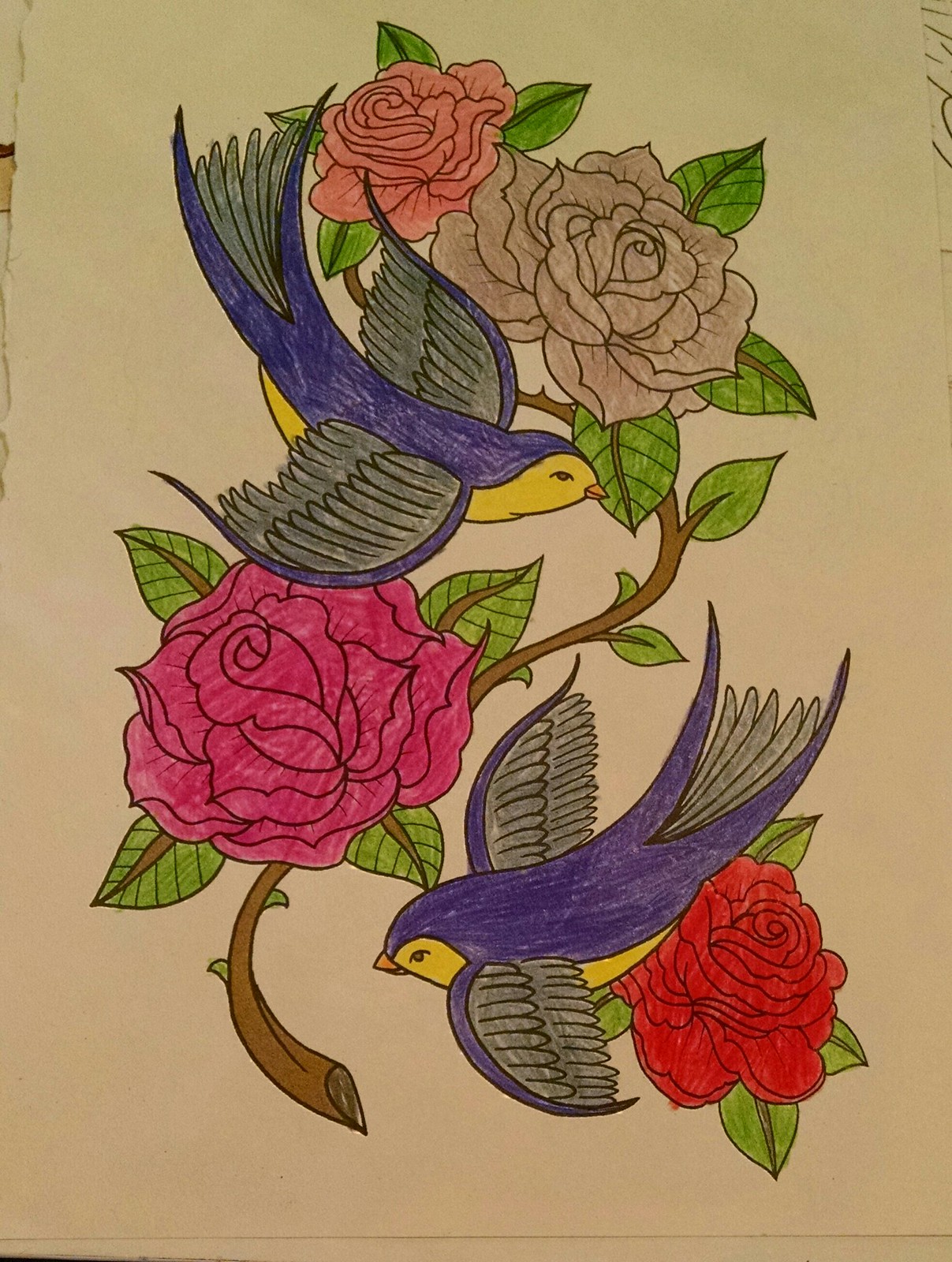This detailed drawing, possibly a page from a coloring book, is rendered on tan paper and depicts a vine of roses flanked by two colorful barn swallows. The scene features four fully bloomed roses in an array of colors: a red rose at the bottom right, adorned with green leaves, a dark pink rose just above it, further up, a gray rose, and at the top, a peach-colored rose. The vine and greenery are meticulously illustrated with green leaves and brown stems.

Each barn swallow showcases a vibrant palette with yellow underbellies and blue backs and wing edges. Their wings and tails are accentuated with gray-green and black feathers, respectively. One bird, perched serenely beside the red rose, has its wings outstretched, displaying detailed feather work. The second bird, also with wings extended, sits between the dark pink and gray roses on the branch. Both birds feature striking black outlines and may have been colored with pencils, adding to the intricate and vivid tattoo flash style aesthetic of the drawing.